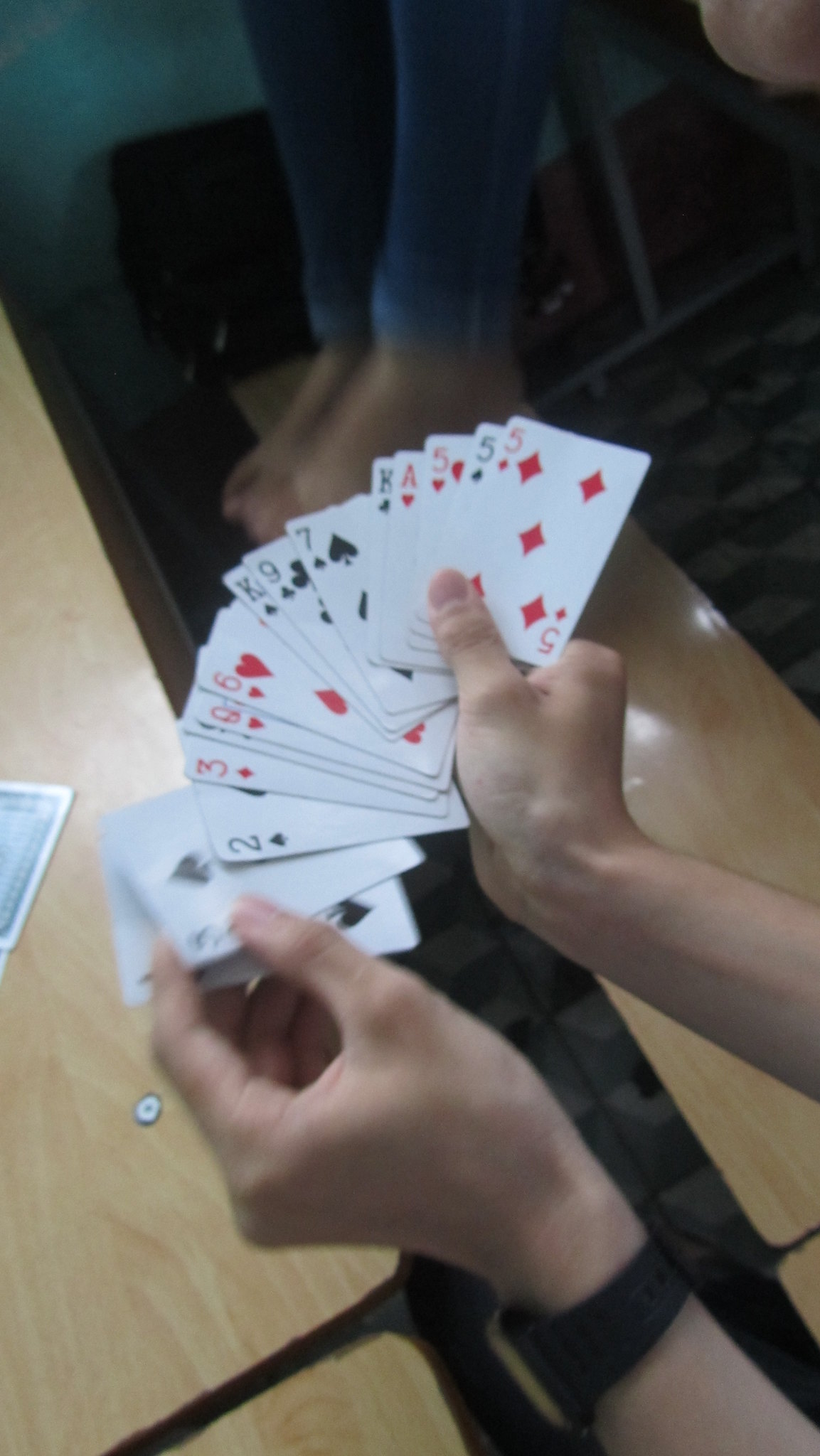In this detailed photograph, a person is captured holding a wide fan of 15 playing cards in both hands, with cards spread out in a striking display. The tall, narrow vertical frame cuts off at their forearms, showcasing only their arms and hands reaching from the lower right corner. The individual, appearing to be white, wears a black wristwatch on the left wrist, indicating a classic style. Their right hand grips the majority of the cards while the left hand pulls out the two leftmost cards, which are slightly blurred, hinting at motion. The cards themselves are from a traditional 52-card deck, featuring a variety of numbers and suits.

The background reveals an indoor setting with a light-colored laminate picnic bench-style table adorned with faux wood grain, positioned in the lower left corner. To the right, the matching bench runs parallel to the table. The legs of a second person seated nearby are visible in the upper right corner, clad in blue jeans with bare feet resting on the bench. The surroundings feature a geometric-patterned carpet in shades of dark gray and tan, creating an illusion of 3D cubes.

On the table lies a single, face-down playing card with a distinctive blue back, adding an element of mystery to the scene. This composition not only captures the act of gameplay but also provides an intimate glimpse into the casual, relaxed environment of the players.